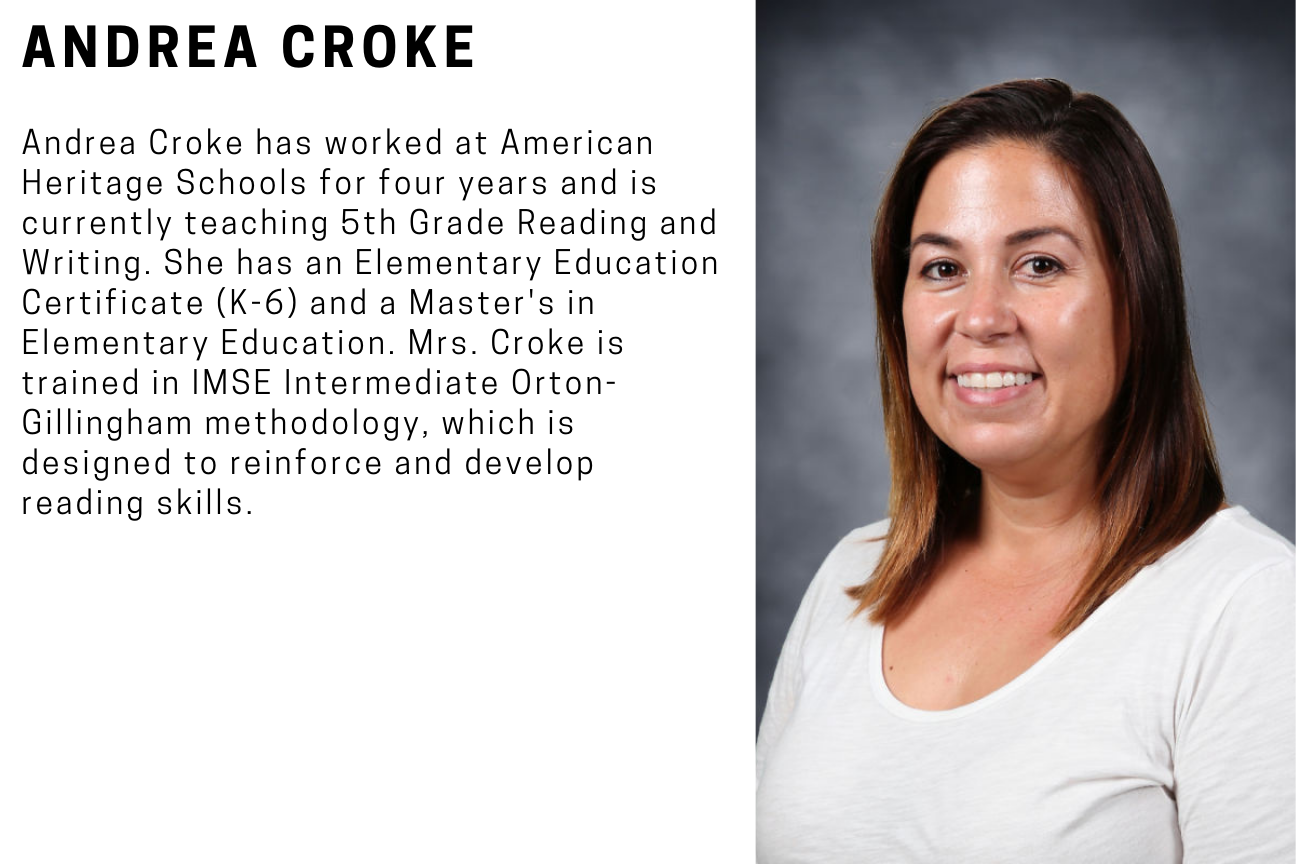The image is an informational clip featuring a biography of Andrea Croak, displayed on the left side with a portrait on the right. The portrait, set against a grayish background, shows Andrea Croak, who appears to be between 35 to 40 years old, smiling and wearing a white long-sleeved shirt. Her dark brown hair falls just below her shoulders. To the left of the image, in bold black capital letters, her name, Andrea Croak, is prominently displayed. Below her name, a detailed paragraph highlights that Andrea Croak has worked at American Heritage Schools for four years and is currently teaching fifth-grade reading and writing. She holds an elementary education certificate for grades K-6 and a master's degree in elementary education. Additionally, Mrs. Croak is trained in IMSE Intermediate Orton-Gillingham methodology, a program designed to reinforce and develop reading skills.